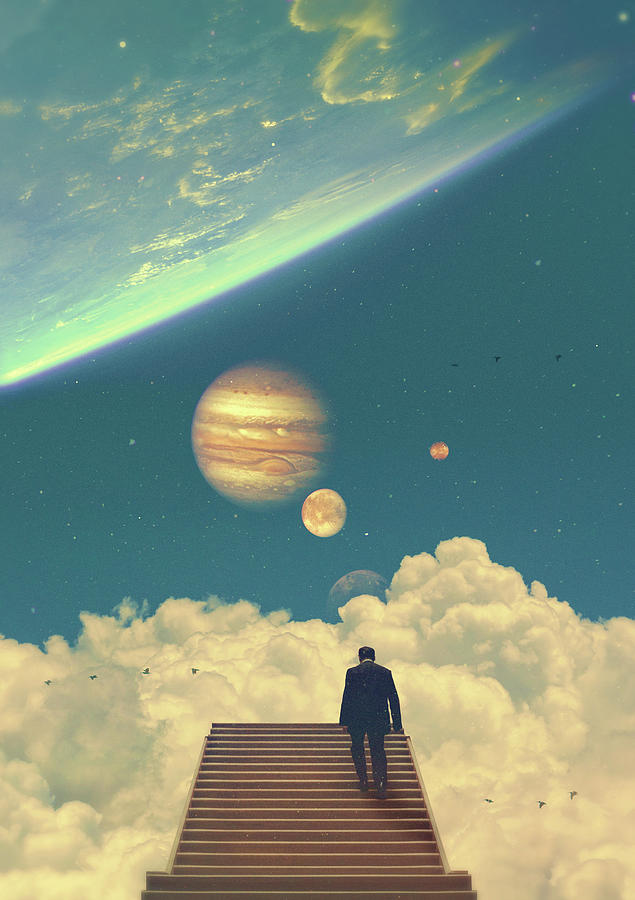The image portrays a highly abstract and surreal scene with a composite of celestial and earthly elements. Dominating the center of the image, a man in a suit, with his back turned, ascends a set of light brown, wooden stairs that lead to nowhere, emphasizing a sense of journey or transition. The suit has a white collar and is slightly blurred and silhouetted, merging enigmatically with the surroundings. 

Situated in space, the bottom portion of the artwork is filled with fluffy white clouds, beneath which dark, starry space extends upwards. Various planets are depicted throughout the piece, such as a large one resembling Jupiter with its distinct brown and light brown bands, a smaller moon of similar hues, a reddish planet possibly Mars, and another indistinct planet blending into the background. Particularly striking is a partial view of Earth in the top third of the image, with its blue surface and white clouds, slightly tilted and spanning from the middle left to the top right.

The sky, a rich shade of dark blue infused with the depths of space, serves as the canvas for scattered white stars and planets. Adding to the surreal quality, several birds are seen flying around the stairs and dispersed across the sky, creating an unusual juxtaposition of terrestrial life in a cosmic setting. The overall style of the artwork is abstract, blending elements of reality with the fantastical expansiveness of the universe.